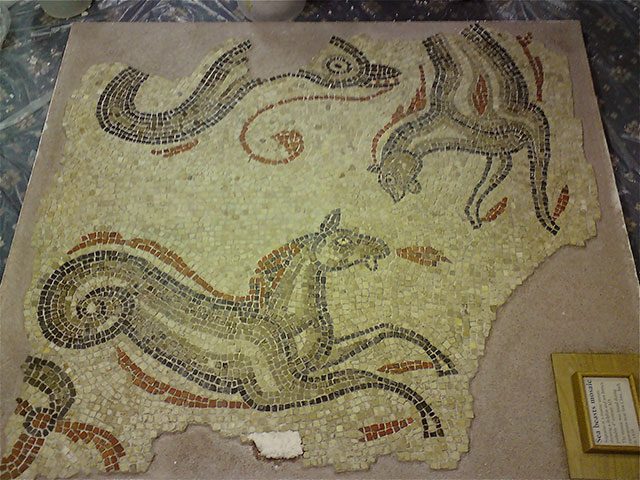The image displays an ancient stone tile, carefully placed on the floor, and accompanied by a wooden placard with some writing in the lower right corner. The tile, likely of ancient origin and housed in a museum, features a mosaic of various creatures. Among them, prominent illustrations depict two horses, and there are elements suggesting a dolphin or possibly a seahorse. The mosaic is composed of extremely small, intricately placed tiles in a palette of greens, blacks, reds, tans, oranges, and whites. The tile is jagged and missing parts, reflecting its age and historical significance. It rests on a tan mat and there are visible jagged and broken edges, adding to its ancient appeal.